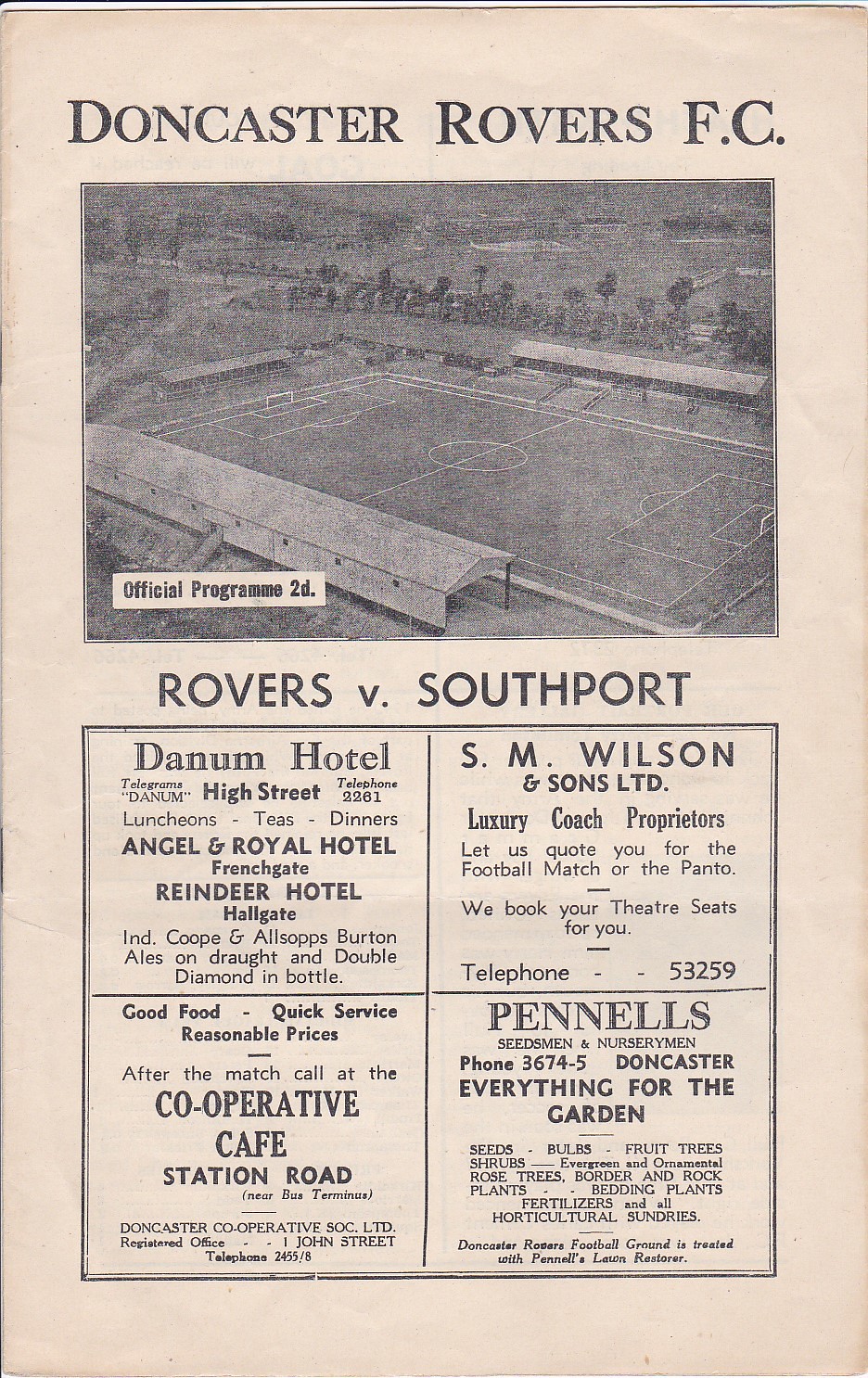This image appears to be a scan of an aged, yellowed page from an old program or magazine. Dominated by a black and white color scheme, at the top of the page, it prominently reads "Doncaster Rovers FC," indicating it is an official program, labeled "2D." The primary visual on the page is an aerial, hand-drawn depiction of the stadium where Doncaster Rovers play, showcasing an empty soccer field (European football) flanked by stands with sheltered open roofs supported by pillars. In the distance, beyond the field, are trees, woods, fields, and buildings. Below the illustration, it states "Rovers vs. Southport," denoting the matchup featured in the program. Further down, four advertisement squares are displayed, listing sponsors: Danum Hotel (promising "Good Food, Quick Service, Reasonable Prices"), S.M. Wilson & Sons, Ltd., Co-operative Cafe Station Road, and Pennells ("Everything for the Garden," offering seeds and shrubs). The entire page, once white, has taken on a yellowed, worn look over time, accentuating its vintage quality.